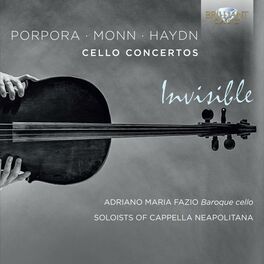The image appears to be an album cover with a black and white, gray-toned background. Prominently displayed at the top in white text are the names "Porpora, Monn, Haydn," indicating the featured composers for the "Cello Concertos." The album title "Invisible" is also included in the design. Dominating the visual is a photograph of an old baroque cello, held horizontally by two hands extending from the left side of the image. At the bottom right, the text reads "Adriano Maria Fazio, Baroque Cello, Soloist of Cappella Neapolitana." The upper right corner features a logo resembling a diamond, adding a distinct touch to the classical aesthetic.